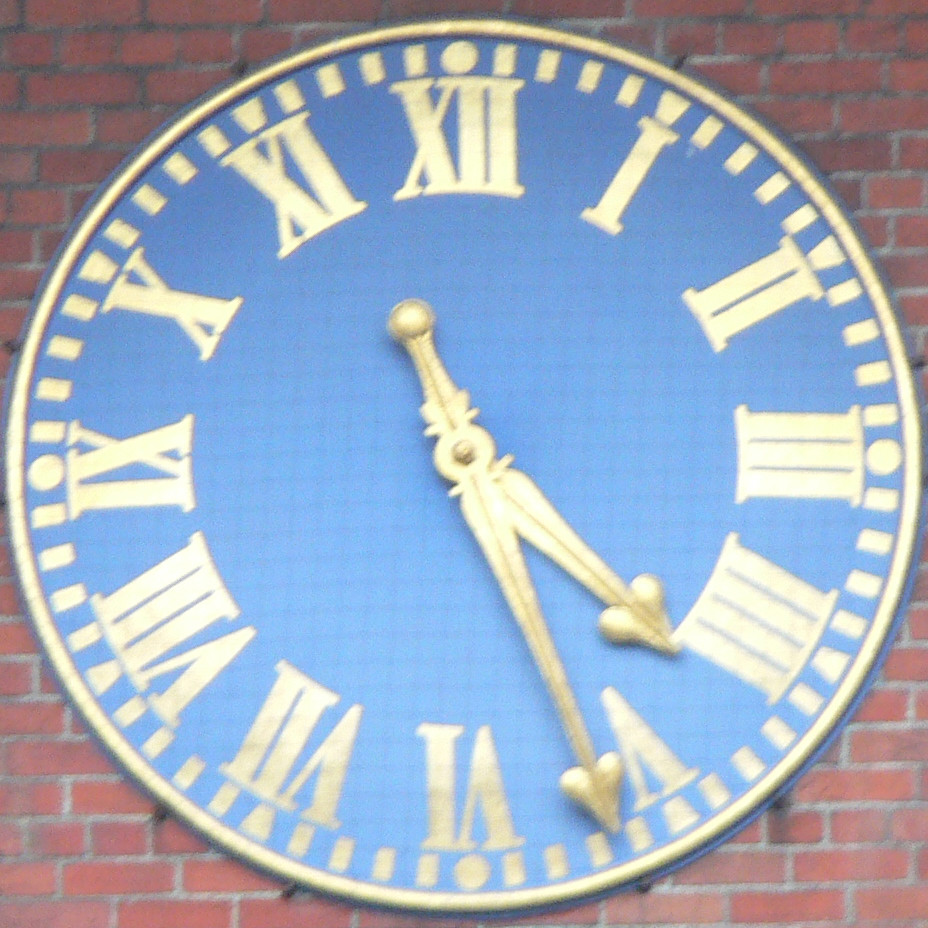A round blue clock with a white border is prominently displayed against a vibrant red brick wall. The clock's design features a unique pattern within the white border consisting of alternating symbols: circle, four dashes, square, four dashes, square, four dashes, and circle, creating a distinctive frame. The inner face of the clock is adorned with Roman numerals, albeit with some inconsistencies: XII, XI, X, IX, VII, VII, VI, V, IIII, III, and I. The time is indicated by two hands; the short hand points slightly past IIII, while the long hand is just past V. A subtle grid pattern is visible within the blue circle, adding an additional layer of texture to the clock's face.